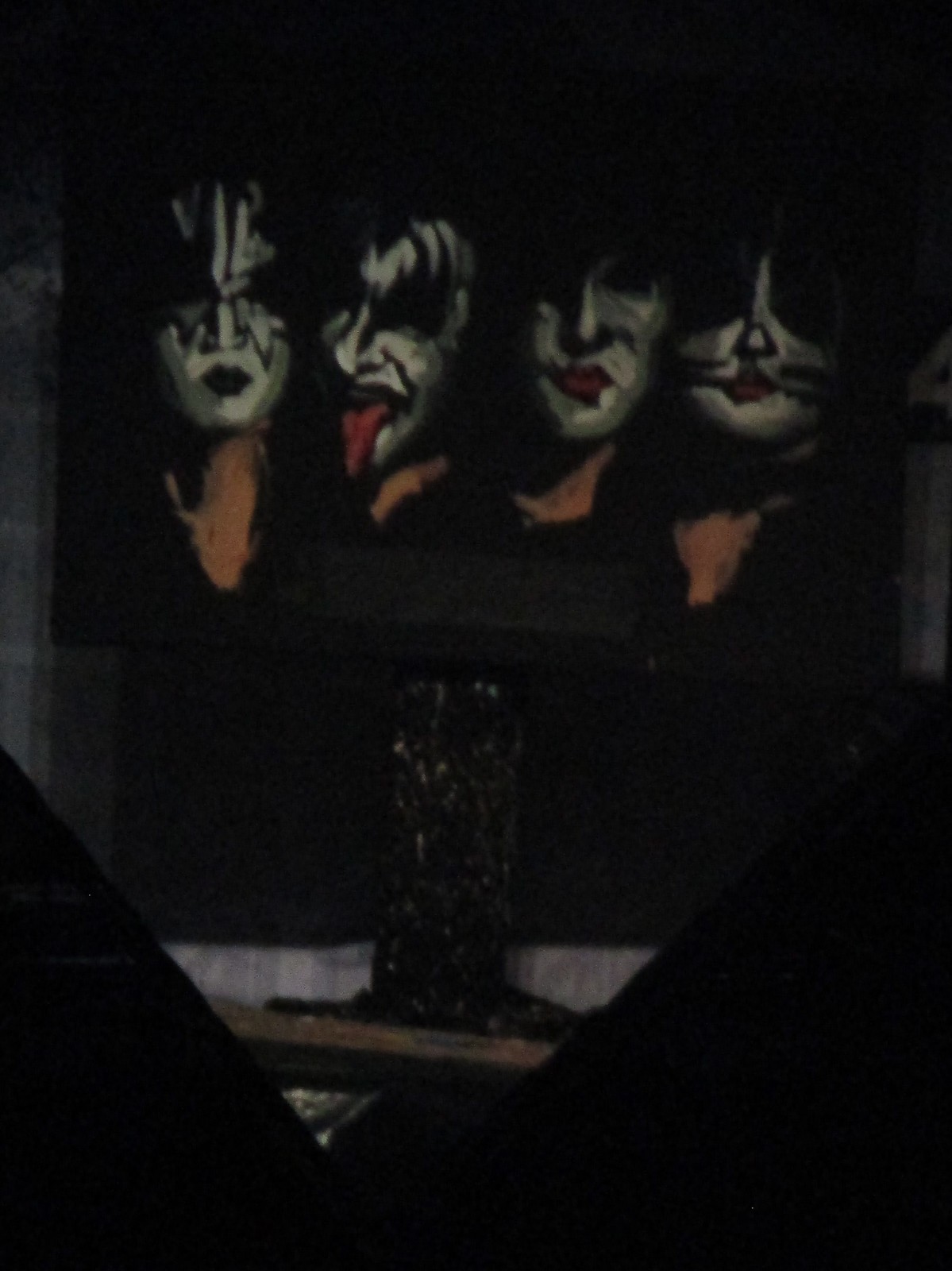This image features a dark, portrait-mode photograph of a painting depicting the legendary rock band KISS. The painting is characterized by its predominantly black background, emphasizing the stark contrast of the members' iconic white-painted faces adorned with distinctive black designs. From left to right, the first member has a stern look with a star around one eye; the second member has his long, serpent-like tongue sticking out, revealing a disturbing intensity; the third member’s face is partially obscured, with red lips that barely emerge from the shadows; and the last member sports whisker-like markings resembling a cat. Their eyes are lost in the darkness, adding to the eerie aura of the image. All members appear topless with visible peach-colored necks and bare chests, their dark attire blending seamlessly into the shadowy background. The painting rests on a wooden stand in a dimly lit room, with subtle details like blue-striped flooring and curtains at the forefront. Overall, this carefully assembled artwork captures the haunting essence of KISS, their theatrical makeup looming out of the void.